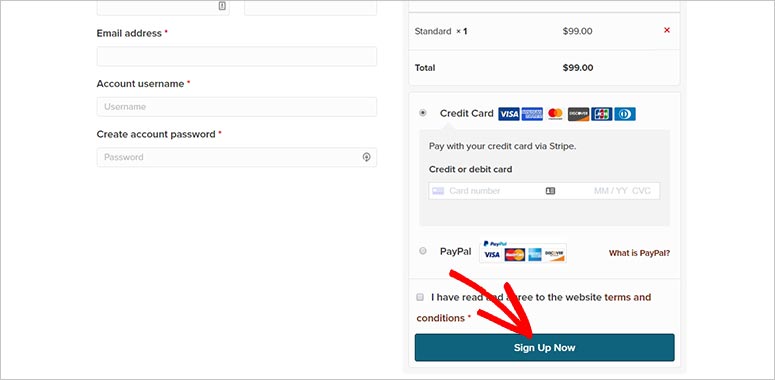The image comprises two sections side-by-side. On the left side, there is a detailed form for creating a new account, including fields for an email address, account username, and a password. The right side showcases the pricing details, stating that the standard subscription costs $99, making the total amount due $99. Below this, there's a section dedicated to credit card information, listing accepted types such as Visa and American Express. Additionally, an arrow is drawn across the image, specifically pointing to a "Sign Up Now" button located at the bottom right corner, emphasizing the call to action.